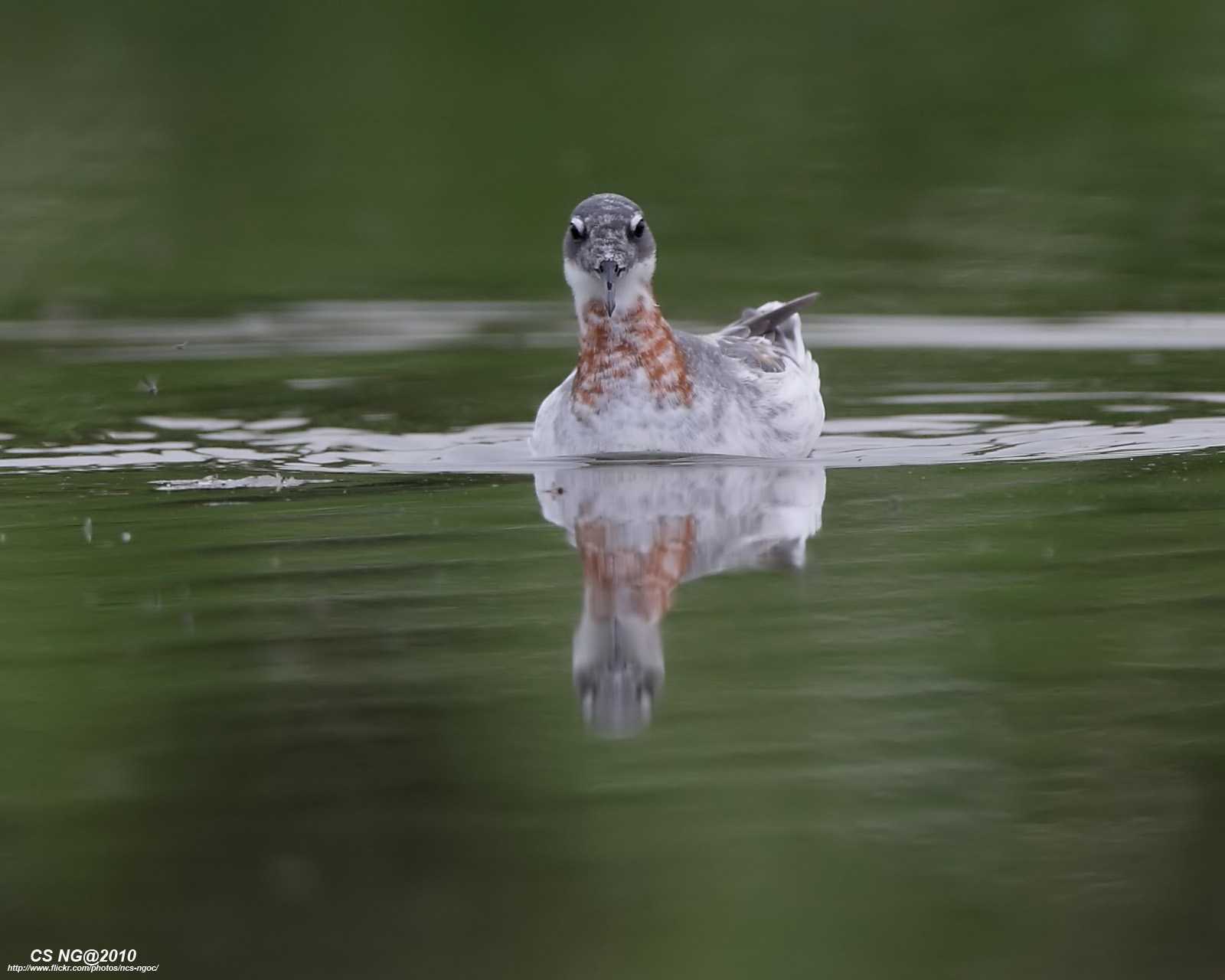This wide rectangular outdoor photograph, taken during daytime in 2010 as indicated by the white font "CSNG at 2010" in the lower left corner, captures a bird in a calm, green body of water with subtle ripples. Darker shadows accentuate the bottom left and right corners of the image, while the top of the photo appears slightly blurred. The green water reflects the bird and a slight upward tilt of light across the center. The bird, which might be a duck or a goose, has distinctive coloring: a small domed gray head, black eyes highlighted by white eyelids, and a delicate, narrow black beak facing down. The upper body features a mix of white and light gray feathers, transitioning into a rust-brown neck and darker gray tail. The fluttering tail and the ripple effect in the water suggest movement. The reflective surface creates a mirror image of the bird directly beneath it, enhancing the visual symmetry.